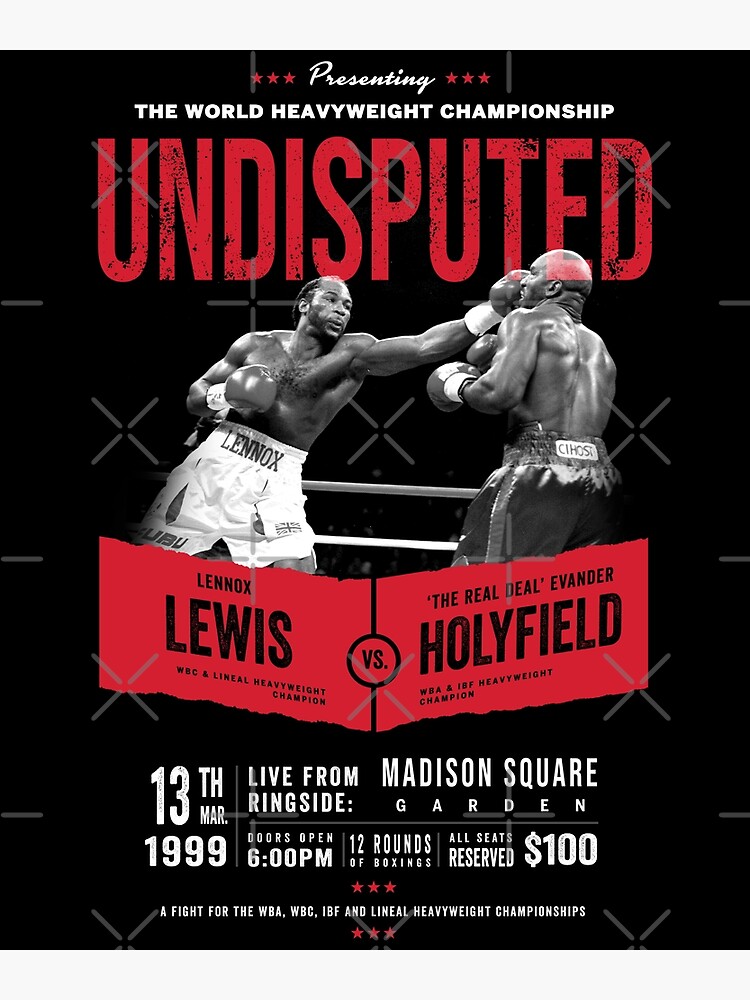Here is a detailed caption for the boxing match poster, combining aspects from all three descriptions:

This vibrant black, white, and red poster announces an epic boxing match for the World Heavyweight Championship. At the top, in bold white letters against a black background, it says "Presenting the World Heavyweight Championship," followed by the word "Undisputed" in large, striking red letters. Central to the poster are two African American male boxers depicted mid-fight: Lennox Lewis on the left and Evander "The Real Deal" Holyfield on the right. Lennox Lewis, WBC and Lineal Heavyweight Champion, is caught in the act of jabbing Holyfield in the face, wearing white trunks with "Lennox" emblazoned on the front. Holyfield, the WBA and IBF Heavyweight Champion, clad in black trunks, recoils slightly from the force of the jab, his left hand positioned near his chest.

Beneath the dynamic imagery, a red banner in black letters spells out "Lennox Lewis versus The Real Deal Evander Holyfield". Below this, in white letters, the event details are prominently displayed: "13th March 1999, live from Ringside at Madison Square Garden," along with specifics such as "Doors open at 6pm", "12 rounds of boxing," and "All seats reserved $100." At the very bottom, additional information emphasizes that this is a fight for the WBA, WBC, IBF, and Lineal Heavyweight Championships.